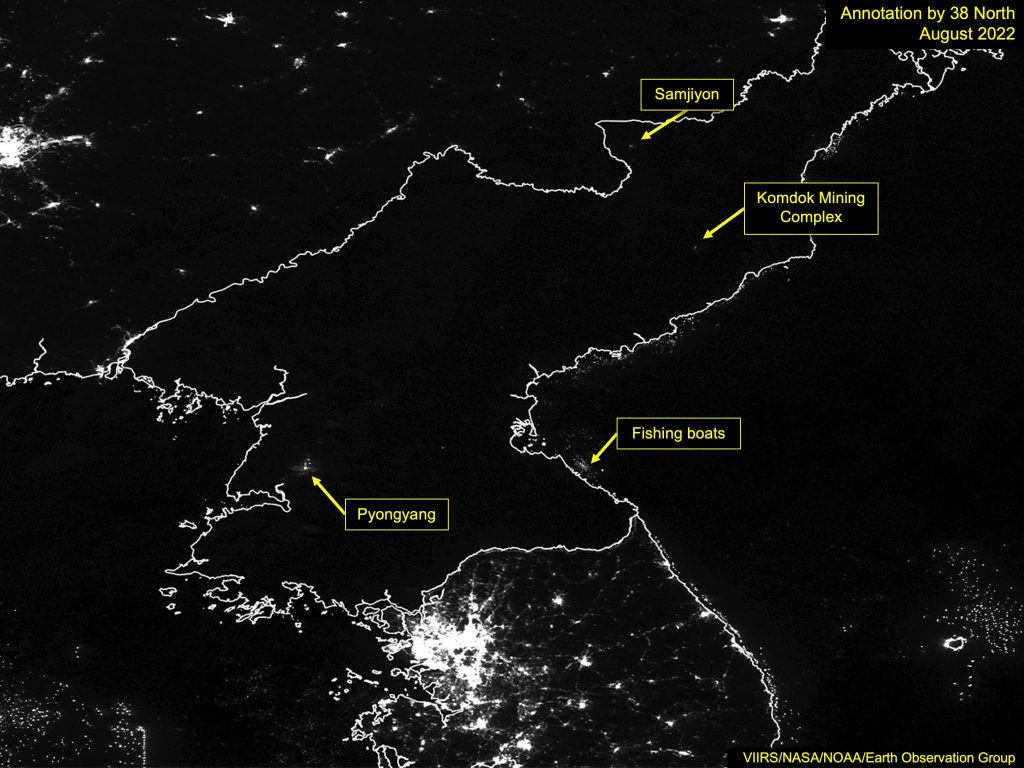This image is an aerial night view of the Korean Peninsula, showing North and South Korea. The image has a black background with white outlining the land, resembling an illustration taken with night vision. Numerous white spots of light are scattered across the map, indicating various points of interest, most predominantly in South Korea and China, which are well-lit compared to the faintly illuminated North Korea. In North Korea, the few visible specks of light are labeled with yellow text and arrows pointing to specific locations: "Samjiyon," "Komdok Mining Complex," "Pyongyang," and "Fishing Boats." Annotations are provided in yellow text, with a remark at the top right corner that reads "Annotation by 38 North, August 2022." Additional credit at the bottom right corner attributes the image to "VIRS NASA NOAA Earth Observation Group." The map highlights the stark contrast in luminosity between the two Koreas and surrounding regions.